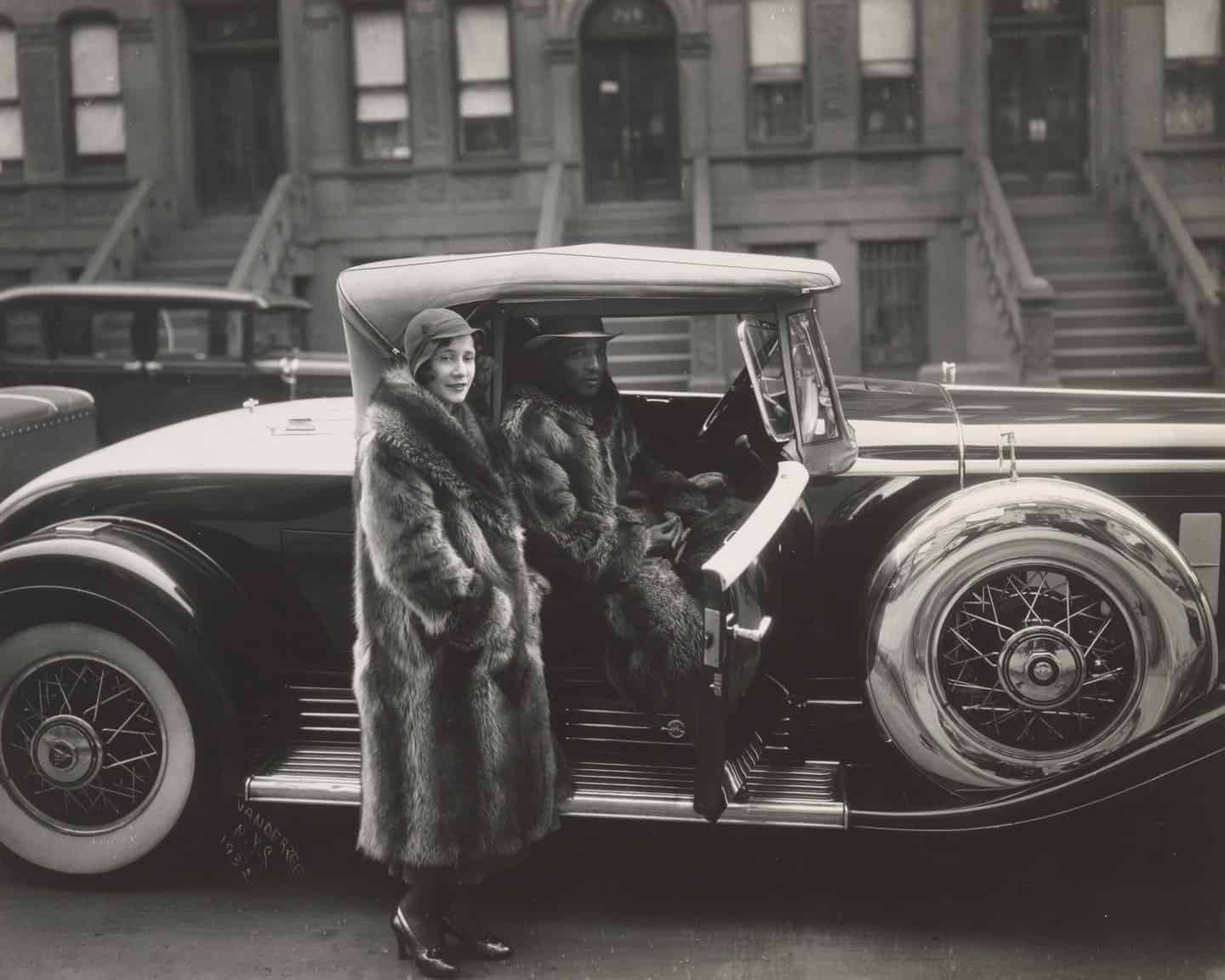This is a vintage black and white photograph of a scene featuring a classic car and two well-dressed individuals, likely taken many years ago. Central to the image is an old-fashioned car, which appears to resemble an early Ford Model T, with distinctive features such as a canvas roof and spare wheels mounted on the front sides, indicating they are not in use. The back wheels of the car have white radial tires, while the front wheels seem to be elevated, possibly due to the car being on a lift.

The photograph is set on a street in front of uniformly connected stone or cement buildings, each with stairs leading up to a raised first floor, suggesting an apartment complex. Two people are prominently featured in the image. Standing to the right side of the car is a woman, dressed elegantly in a large fur coat, high heels, and a hat with a very short brim. Sitting inside the car, in the passenger seat with the door open, is an African man. He is also wearing a long fur coat and a brimmed hat.

In the background on the left, another old-style car can be seen, adding to the historical ambiance of the photograph. This detailed composition hints at an urban setting, possibly in a large city like New York City. The overall scene captures a glimpse into a bygone era, showcasing fashion and automobile design characteristic of the time.